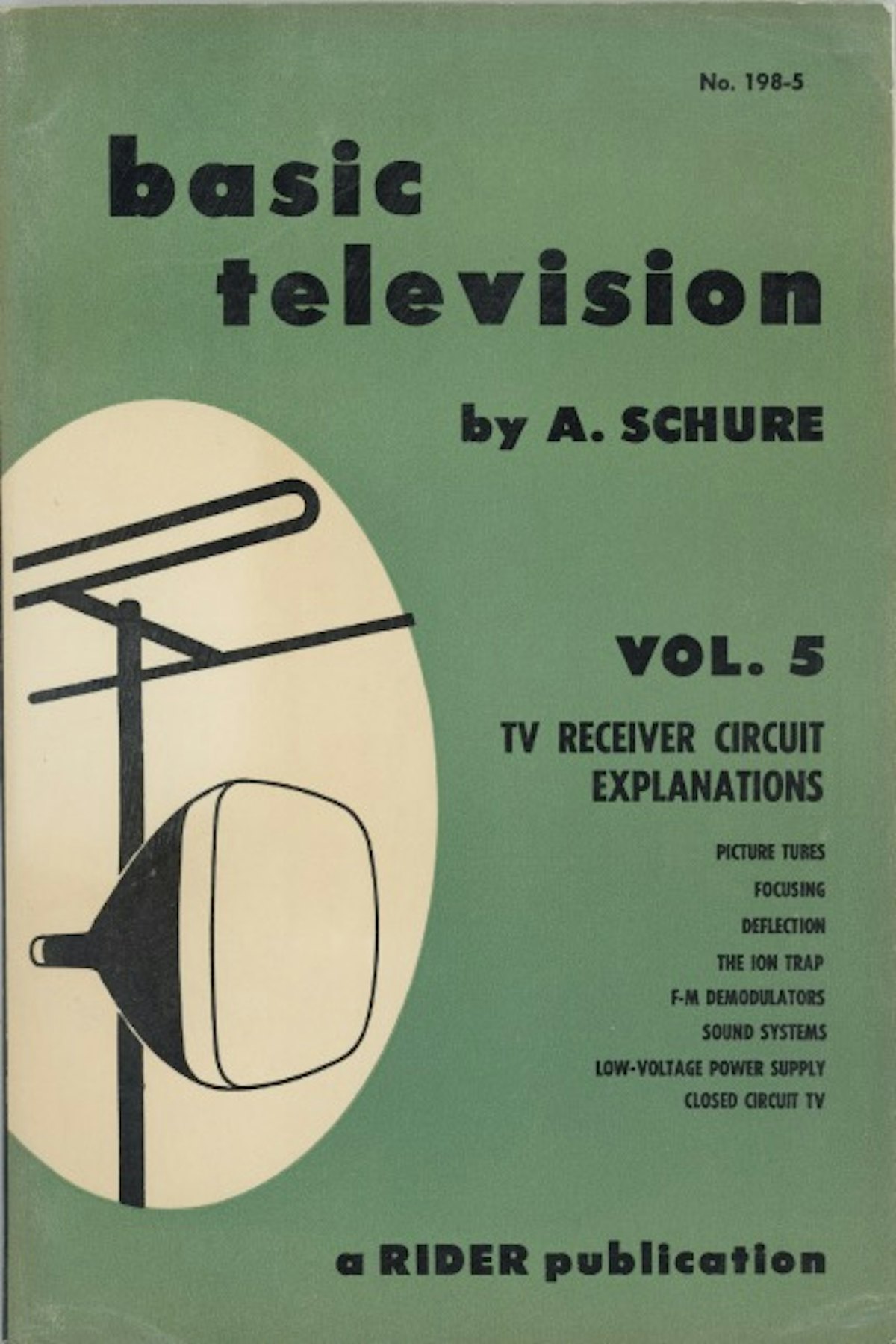The cover of the book, which appears aged and dingy with a faded olive green background on beige paper, features a simple black font with its title and details. In the upper right corner, it is labeled with the number 198-5. Centered beneath that, the title "basic television" is written in lowercase, followed by the author's name, "A. Schur." Further down, it specifies "Volume 5, TV Receiver Circuit Explanations," and includes additional sections: Picture Tubes, Focusing, Deflection, The Ion Trap, FM Demodulators, Sound Systems, Low Voltage Power Supply, and Closed Circuit TV. Towards the bottom left, it says "A Writer Publication." On the left side of the cover, there is a beige oval shape enclosing a black outline drawing of a TV receiver antenna, featuring one traditional antenna at the top and a parabolic-grade antenna near the center, mounted on a pole with wires extending across.